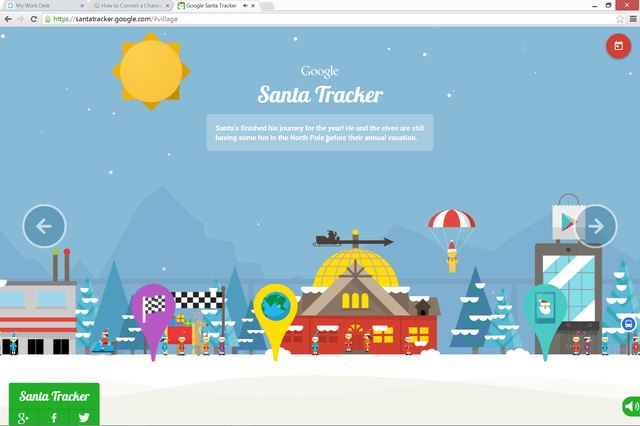This screenshot captures a vibrant and interactive section of the Google Santa Tracker website. Displayed in landscape mode, the Chrome browser reveals three tabs: the first labeled "My Desk," the second "How to Convert Something," and the active tab displaying "Google Santa Tracker" with the URL santatracker.google.com.

The central focus of this image is a digital artwork created by Google, featuring a whimsical, night-blue sky dotted with a bright sun in the upper right corner, its rays pointed sharply downward. Below, a charming village stretches across the scene, complete with houses, a race finish banner, and a weathervane shaped like Santa Claus. Amidst the village, a Santa figure appears to be descending by parachute near what seems to be Santa’s factory and the Google Play Store icon.

Navigation arrows on either side of the scene indicate that users can browse through additional images. Prominently displayed text reads, "Google Santa Tracker: Santa's finished his journey for the year. He and the elves are still hunting some fun in the North Pole before their annual vacation." In the lower left corner, the Santa Tracker logo appears in green, enhancing the festive theme.